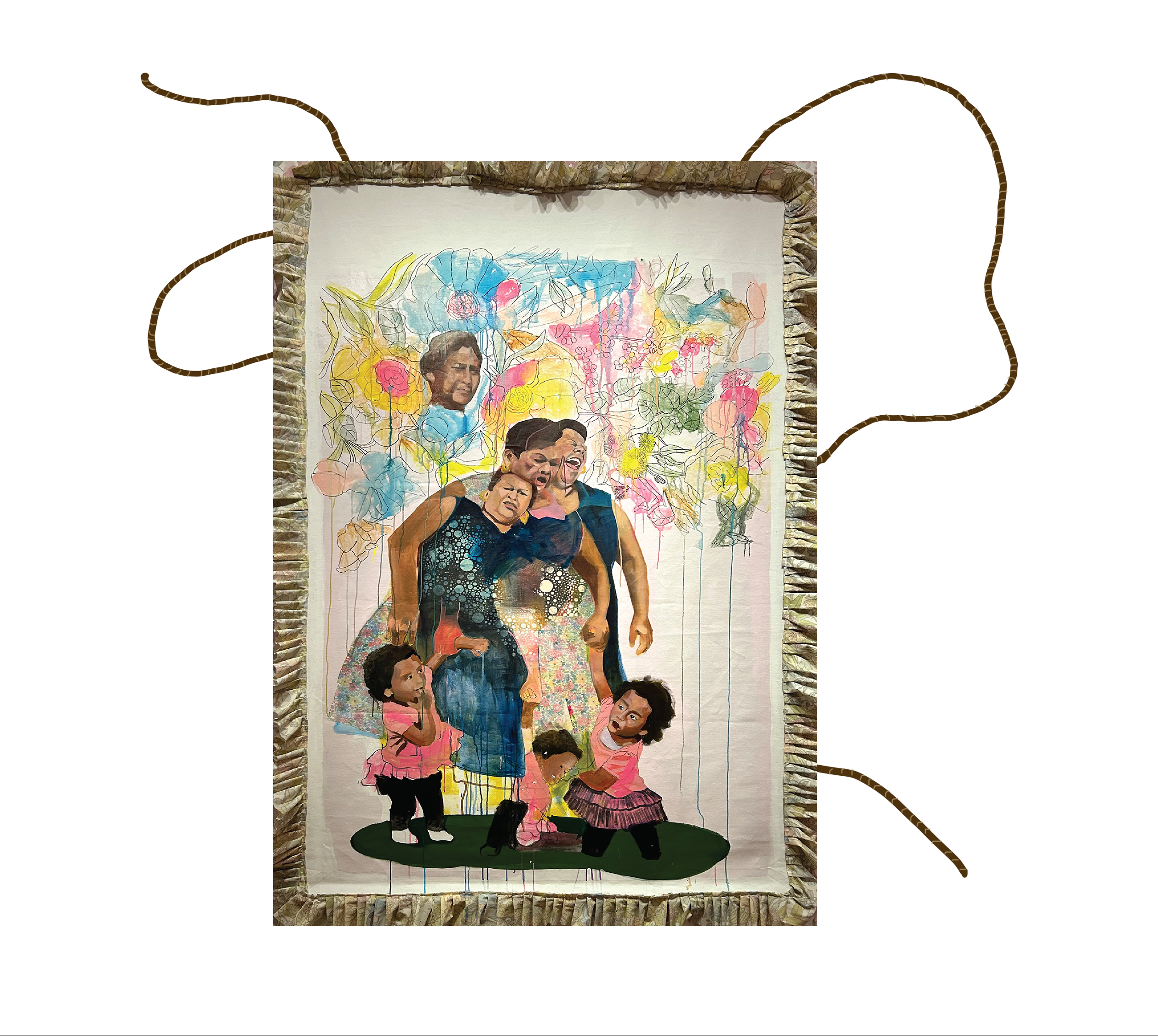In the image, set against a white background, there appears to be a highly textured painting encapsulated within a wooden frame. At the top of the image is an inset portrait of a woman amidst a vibrant clutter of flowers in yellow, pink, and blue hues. Below this inset, a family group is depicted.

At the center, there is a woman with short, sleeveless blue dress. Her black hair matches those around her, and she is leaning into another woman beside her. This woman similarly has bare arms and a blue dress. To the right is a man who appears to be laughing. Interwoven into this familial scene are three young children, dressed in pink dresses with black leggings, some likely around one or two years old. They stand on an indistinct green area, perhaps meant to resemble a golf course. The tallest child is holding the central woman's hand, infusing the image with familial warmth and joy.